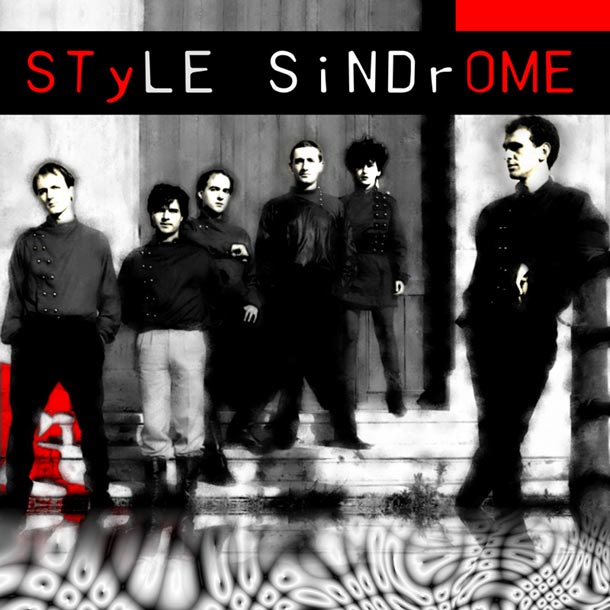This image, likely an album cover titled "Style Syndrome," features a square layout with a predominantly gray background, incorporating varying shades of gray along with red, black, and some silver. At the top of the cover, the text "Style Syndrome" is prominently displayed. The upper left-hand corner has a vertical strip of light gray, while the middle portion contains a vertical strip of dark gray that resembles a wood fence. The upper right-hand corner transitions from a vertical strip of red down into light gray.

Central to the image are six individuals standing on white steps in front of a large door, surrounded by a swirling, faded backdrop with abstract shapes. From left to right:

1. The first person, a man, stands on the ground wearing black pants and a long-sleeve black shirt, with short brown hair.
2. Next to him is another man in light-colored pants and a black shirt, featuring short dark hair with bangs over his eyebrow.
3. The third person, whose body is partially obscured, rests his arm on the shoulder of the person to his left and has short brown hair.
4. The fourth individual is a man dressed in all black with short brown hair.
5. To his right seems to be a woman with short black hair, wearing a dress with leggings and blurred-out shoes.
6. On the far right, another man is leaning against a wall, legs crossed, dressed in all black with short dark hair.

The overall design suggests an artistic and modern aesthetic, potentially serving as the cover for a music album or other creative work.